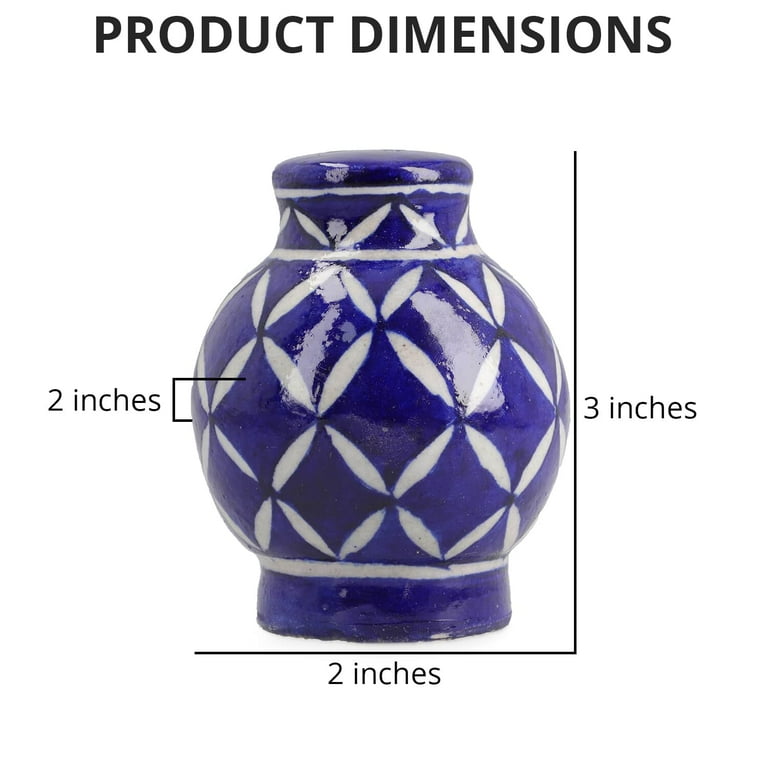This image showcases the product dimensions of a ceramic item, potentially a vase or a small urn. At the top, the text "PRODUCT DIMENSIONS," written in black, plain font, indicates the dimensional details of the item. The ceramic piece features a glossy, deep royal to navy blue surface adorned with a white pattern that resembles flower petals forming diamond shapes. The object is spherical in the middle with a slightly curved top and a stable base. The dimensional markings show it as 3 inches tall, 2 inches wide, and 2 inches in diameter. These measurements are indicated by lines on the right and bottom of the image, forming a right angle, with the vertical line representing the height and the horizontal line the width. The white pattern includes a distinctive feature of four petals creating a blue diamond shape, and there are white rings just above the base and near the top.